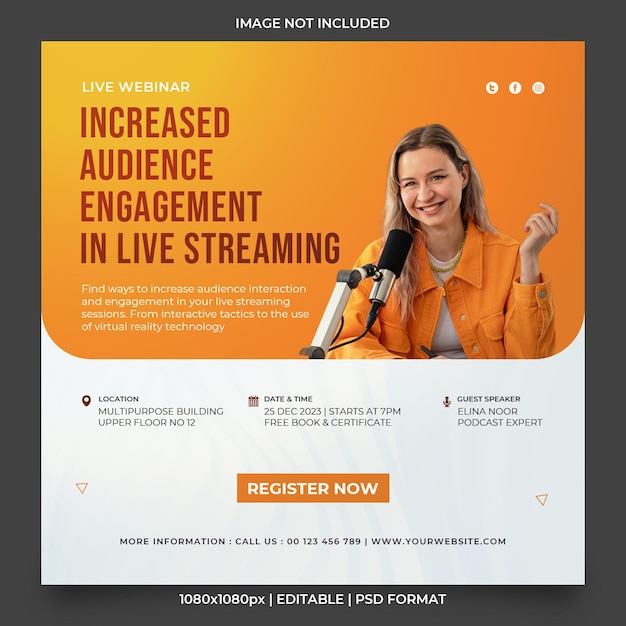This image is a detailed advertisement for an in-person live webinar focused on increasing audience engagement in live streaming. The event is hosted by Alina Noor, a podcast expert, and is scheduled for December 25th, 2023, at 7 p.m. in the multipurpose building, upper floor, number 12. The ad prominently features a smiling woman with light brown or blonde hair, wearing an open orange jacket over a white shirt and a necklace, with a microphone in front of her. The background is orange, harmonizing with her outfit. 

Text elements include the main message, "Live Webinar: Increased Audience Engagement in Live Streaming," in large dark red letters, with smaller white text above it stating "Live Webinar." There's a subtitle offering details about the webinar's content, including strategies for boosting interaction through interactive tactics and virtual reality technology. Social media icons for Twitter, Facebook, and others appear in the upper right corner. Three outlined sections in the middle provide specific details: the location, date and time, and guest speaker. The ad highlights a free book and certificate for attendees. An orange "Register Now" button is featured prominently, along with contact information and the website, yourwebsite.com. Despite its professional look, the presence of the template URL suggests it might not be a real ad.